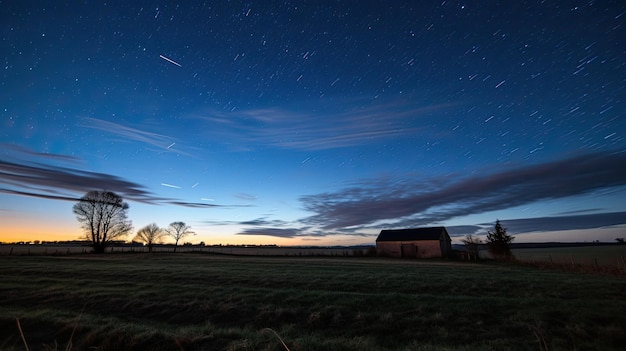In this nighttime photograph, a building, likely a barn, stands amidst a vast, flat expanse of grassy land or farmland under a darkening sky. The sky dominates about 70% of the image, transitioning from a dark black at the top to a deep blue as it descends. At the horizon, a thin band of orange suggests a recent sunset. Wispy gray clouds extend across the sky, converging towards the center, enhancing the time-lapse effect created by thin streaks that resemble falling stars. To the right of the central building are a couple of trees, while on the left side, three tree shapes are discernible. Despite the darkness, the scene is detailed with the building's roof appearing almost black and its walls a brownish color. The land around it is a dark green, nearly black, making it difficult to identify specific crops or grass. Overall, the image captures the serene yet eerie beauty of a rural landscape transitioning into night.